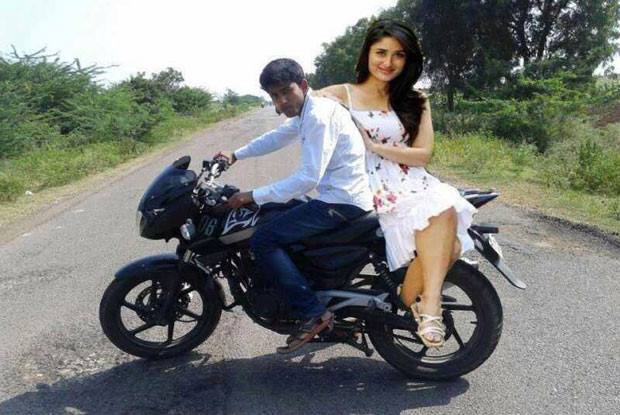In this image, we observe a young couple positioned on a black motorcycle, which is parked sideways in the middle of an asphalt road. The backdrop features lush greenery with various trees, bushes, and vegetation, indicating a countryside setting. The day is bright and sunny with a clear, cloudless sky.

The man, who appears to be of Indian descent, has dark skin and black hair. He is dressed in a white, long-sleeve polo shirt, blue jeans, and sandals with black straps and brown bottoms. He is seated at the front of the motorcycle, gripping the handlebars with a serious expression on his face, as if preparing to ride.

Behind him, a woman with long dark hair sits sideways on the motorcycle, facing the camera. She is dressed in a white spring dress adorned with a delicate floral pattern, possibly featuring small red flowers, and wears white sandals. Her smile is bright and engaging, adding a joyful touch to the scene.

Despite the idyllic setting, there is a suggestion that the image might be photoshopped; the size disparity between the man and the woman appears unnatural, possibly indicating that the woman was superimposed onto the image.

The motorcycle itself is black and features the number "06" on the front. The overall scene creates a picturesque snapshot of the open road, freedom, and a sunny day, albeit with a hint of digital alteration.